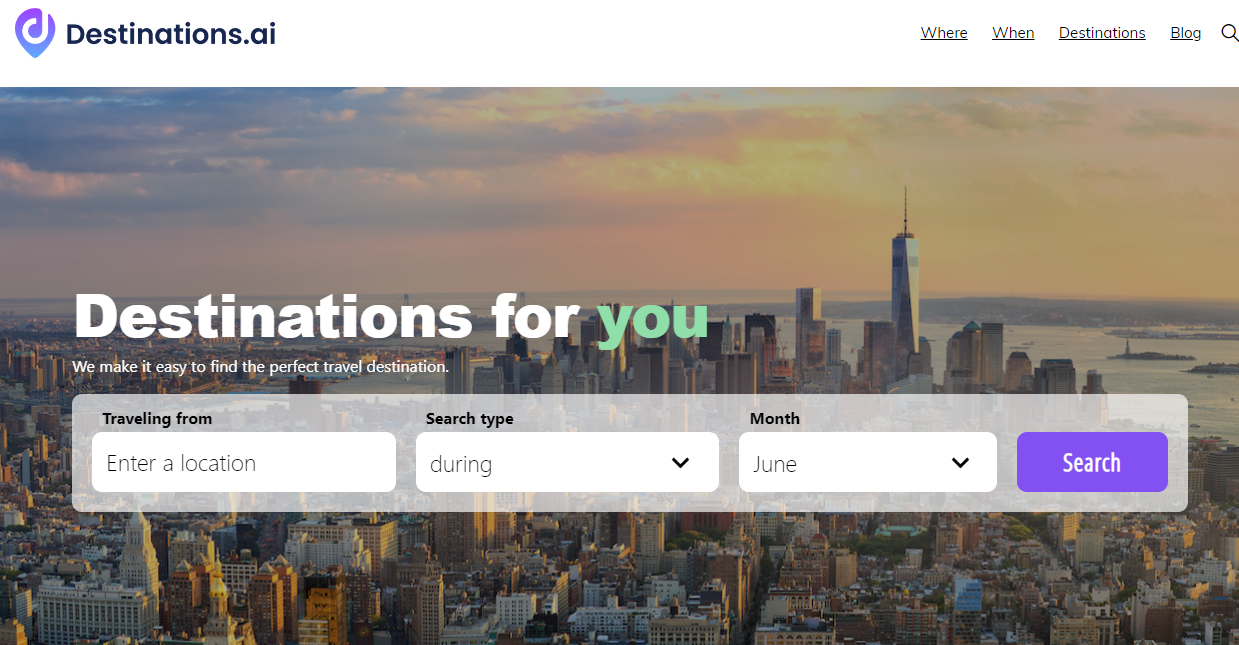The image features a sleek, modern webpage design. In the upper left corner, a bi-color purple and blue location icon emblazoned with the letter 'D' is prominently displayed, accompanied by the text "Destinations.ai". To its right, a horizontal navigation bar presents options labeled "Where", "When", "Destinations", "Blog", and an icon resembling a magnifying glass, symbolizing search functionality.

Below the navigation bar, the header "Destinations for You" is displayed, followed by a tagline: "We make it easy to find the perfect travel destination." A search box beneath this tagline offers fields for users to input their current location ("Traveling from") and specify the "Search type" and "Month." The interface also incorporates a purple search button, while other buttons remain white, maintaining a clean aesthetic.

The background of the webpage offers a picturesque view of Manhattan at dusk, likely around 5 to 7 PM. The scene captures the setting sun casting a warm glow over numerous towering skyscrapers and buildings, emphasizing the bustling city's iconic skyline.

Overall, the webpage presents a straightforward and user-friendly design with a consistent color scheme, predominantly featuring white and black text, except for a highlighted word in green, adding a touch of distinction. The layout is both simple and visually appealing, guiding users effortlessly through the travel search process.